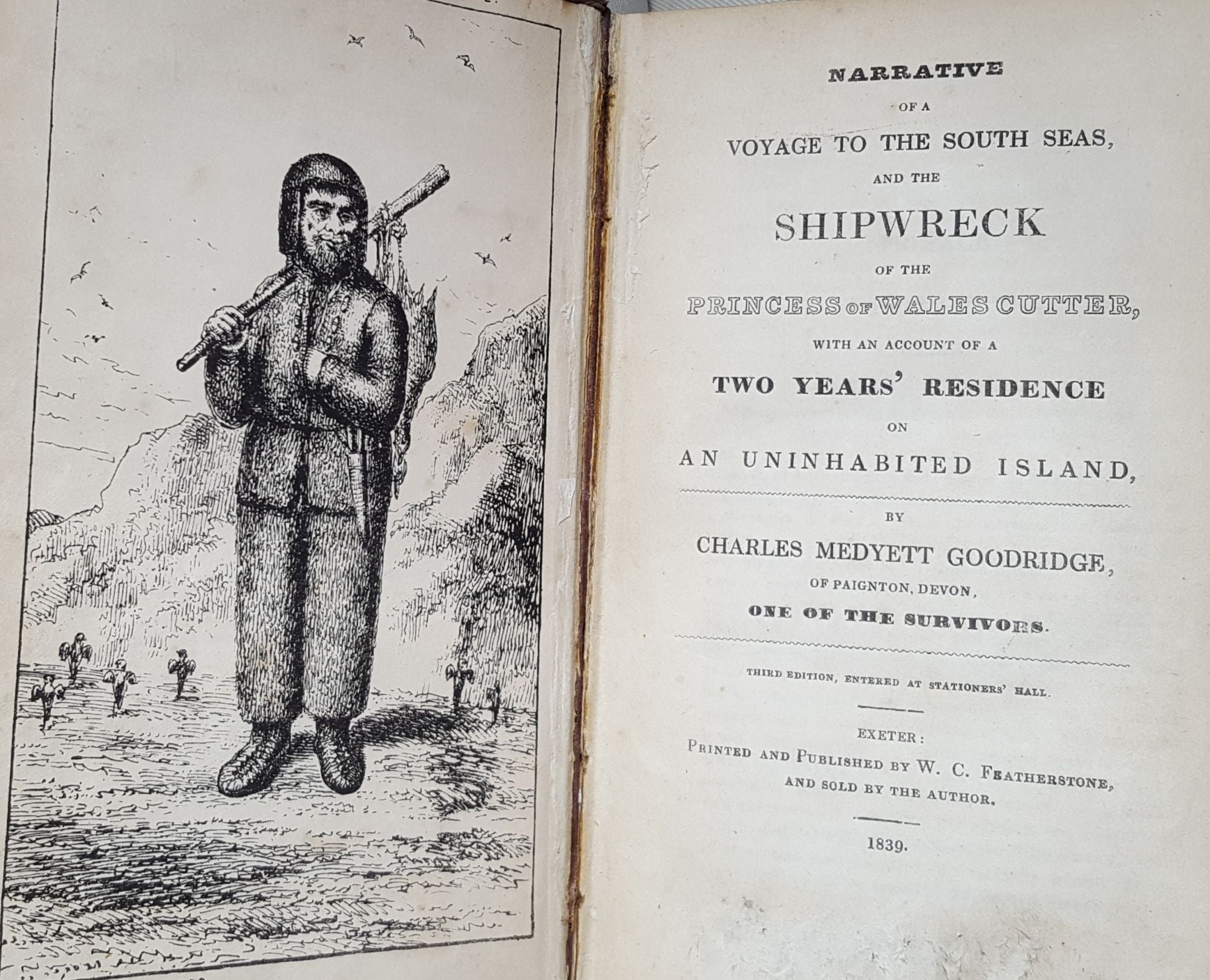The image depicts an old, tattered book, possibly from the 1800s or early 1900s, featuring a detailed illustration on the left page and text on the right. The left page has an ink drawing bordered by a rectangular frame. The illustration shows a mountainous, hilly landscape with fine lines suggesting grass, shadows, and several small cacti or trees. A man, likely around 30, dressed in a fur jacket and pants, stands in this landscape. He has a hood over his dark hair and a knife hanging from a belt around his waist. His right arm is bent at the elbow, holding a stick resting on his shoulder, with two birds hanging from it. His left hand is inside his jacket, and he has a slightly satisfied expression on his face. The right page features centered text in various fonts and sizes. At the top, in bold, it reads "NARRATIVE," followed by "Voyage to the South Seas" and "Shipwreck." Further down, it mentions "Princess of Wales, Cutter," details an "account of two years' residence on an uninhabited island," and credits "Charles Mediat Goodridge of Paignton, Devon, one of the survivors." At the bottom, it states, "Entered at Stationers Hall, Exeter, printed and published by W.C. Featherstone, and sold by the author, 1839." The book is primarily in shades of black, white, gray, and brown, emphasizing its aged and worn condition.